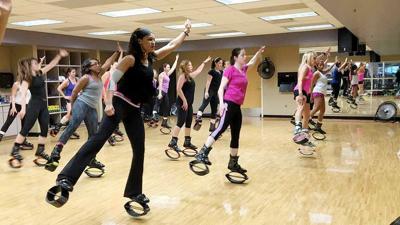The image depicts an exercise class taking place in a studio with a wooden floor. There are approximately 15 women arranged in lines, all engaged in synchronized movement. Each woman is balancing on a pair of unusual shoes equipped with hollow, oval-shaped springs on the bottom, suggesting they are designed for bouncing or adding a level of resistance. The participants have their weight on their left legs, with their left arms extended upward and their right legs kicked out to the side. They appear focused and in unison, seemingly transfixed by something out of the frame. The setting includes a mirror in the background, indicating a dance studio or small gymnasium, and the image itself is of relatively low quality. There is no text on the photo, and the ambiance reflects typical studio colors and design.